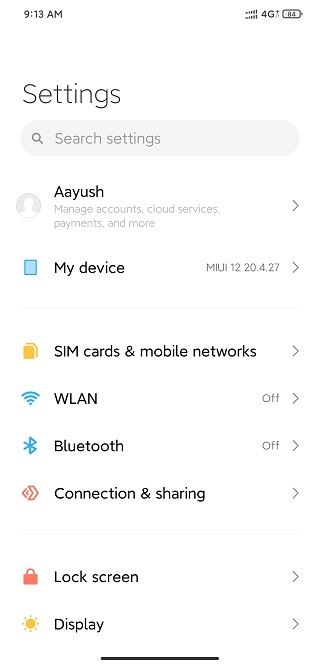This detailed image shows the settings menu of an electronic device. At the very top, the word "Settings" is prominently displayed in bold black lettering. Directly beneath the title is a search bar, allowing users to search for specific settings within the menu.

Just below the search bar, there is a section labeled "Ayush," spelled A-A-Y-U-S-H, which provides access to manage accounts, cloud services, payments, and other user-related settings.

Moving down, next to a small blue square icon, is the "My Device" section, indicating MIUI version 12.20.4.27. Underneath "My Device," there is a yellow square icon resembling a SIM card, labeled "SIM Cards and Mobile Networks."

Further down, there is a section titled "WLAN," indicating Internet settings, with a current status of being off. Below this, there is a Bluetooth symbol accompanying the word "Bluetooth," which is also turned off. 

Following this, the next category is "Connection and Sharing." 

At the very bottom of the screen, an icon of a lock symbolizes the "Lock Screen" settings, and beneath that is a small sun icon paired with the word "Display," indicating display settings options.

This image effectively captures the full range of settings available on the electronic device, organized in a clear and structured format for easy navigation.